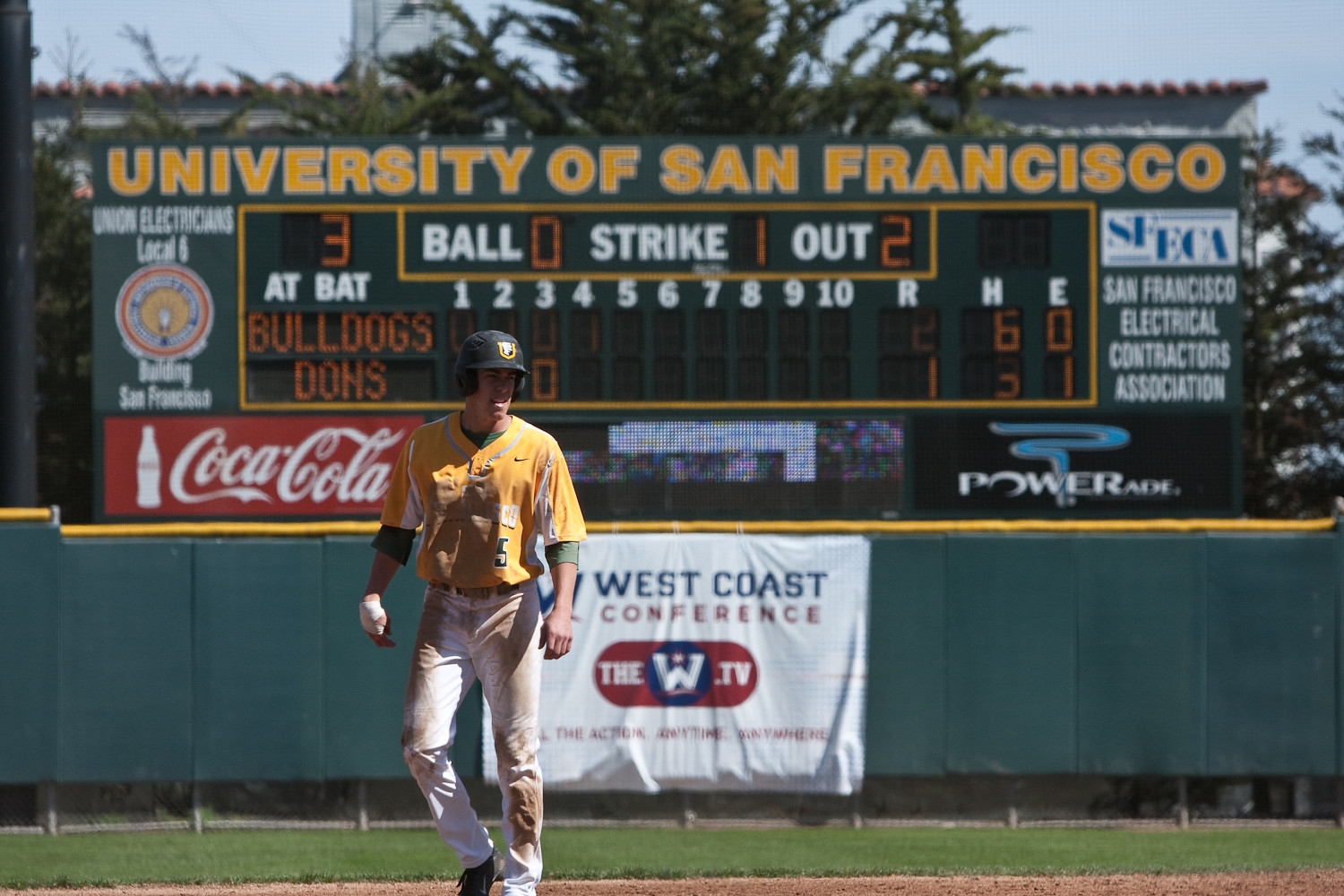This is a detailed outdoor photograph taken on a clear overcast day featuring a man standing on a baseball field. He is dressed in a yellow short-sleeved jersey with a Nike symbol and the number 5, paired with white pants that are dirty, and a black baseball hat. His right hand is wrapped up, indicating he has either a glove or a bandage, and dust covers his clothes, suggesting he has been playing. The green grass of the field and the surrounding dirt are visible in the scene.

In the background, the scoreboard prominently displays "University of San Francisco" in yellow letters against a green backdrop. It shows a score with various details: "At bat: 3," "Bulldogs vs Dons," "Ball: 0," "Strike: 1," "Out: 2," with a sequence of numbers indicating runs, hits, and errors. There are multiple advertisements on and around the scoreboard: the "San Francisco Electrical Contractors Association" and "Union Electricians Local 6, building San Francisco" appear on the sides. Below the scoreboard, there are advertisements for Coca-Cola and Powerade, along with banners reading "West Coast Conference" and "The W.TV - The action anytime, anywhere." The sky and some trees are also visible, enhancing the outdoor setting of this dynamic image.